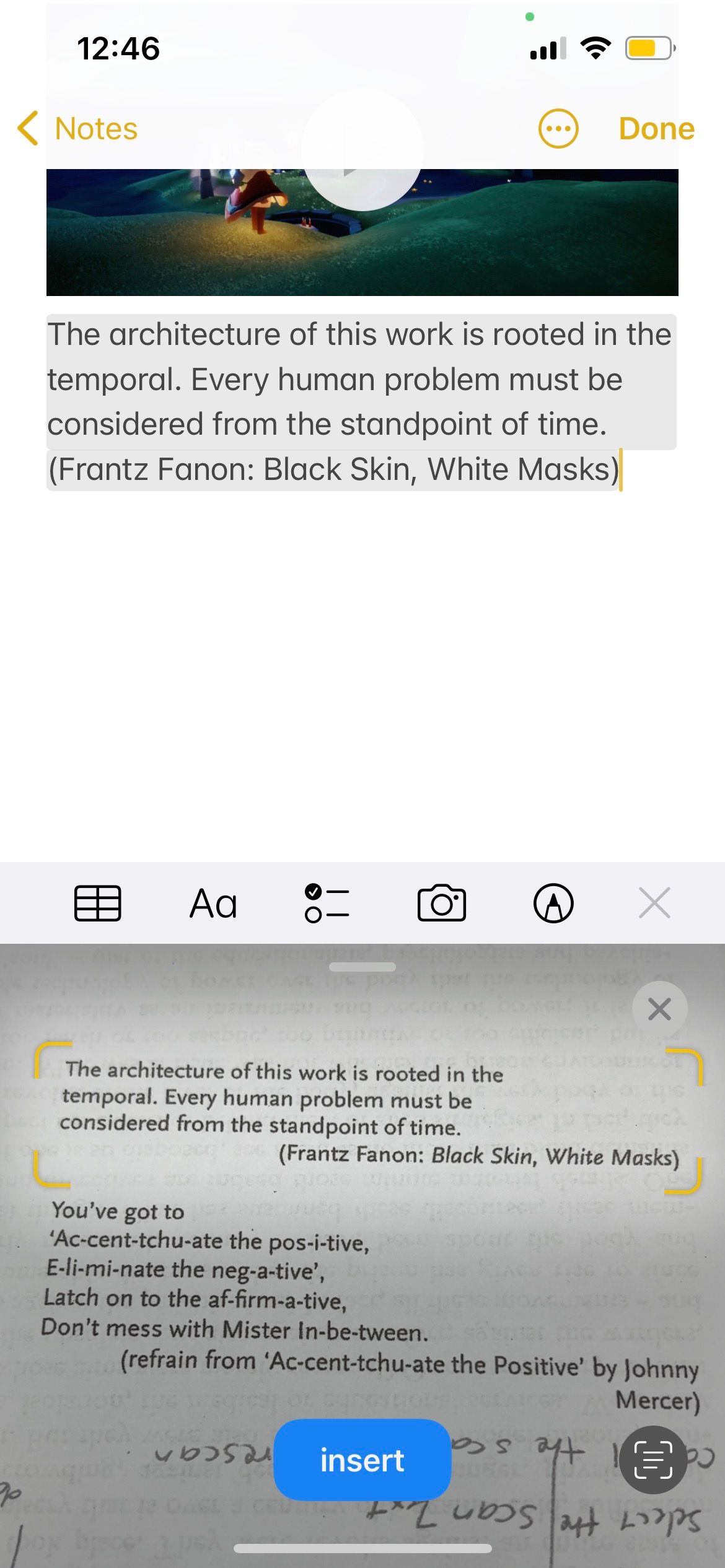**Detailed Caption:**

This is a screenshot taken on a vertical, portrait-oriented smartphone. The top bar of the phone displays the time as 12:46, accompanied by a service indicator, a Wi-Fi signal icon, and a battery icon showing a level slightly above half. Below this top bar, a user interface is visible with a 'Notes' button and a 'Back' button on the left, a 'More Options' button represented by three vertical dots, and a 'Done' button on the right. 

The main content of the screenshot captures an article excerpt which reads: "The architecture of this work is rooted in the temporal. Every human problem must be considered from the standpoint of time. – Frantz Fanon, Black Skin, White Masks." This text suggests an analysis or description of a piece of artwork or a painting.

Further down, the interface features icons for font customization, picture upload, lighting options, etc. Below these icons, an image of a document is partially visible, which appears to repeat the text quoted in the article.

Additionally, beneath the text and image, there is a quotation: "You've got to accentuate the positive, eliminate the negative, latch on to the affirmative, don't mess with Mister In-Between," followed by "Refrain from Accentuate the Positive by Johnny Mercer." Handwritten notes can be seen below this quotation, with an 'Insert' button centrally located within this section.

This detailed observation highlights the various elements present in the screenshot, offering a clear description of the content captured on the phone.